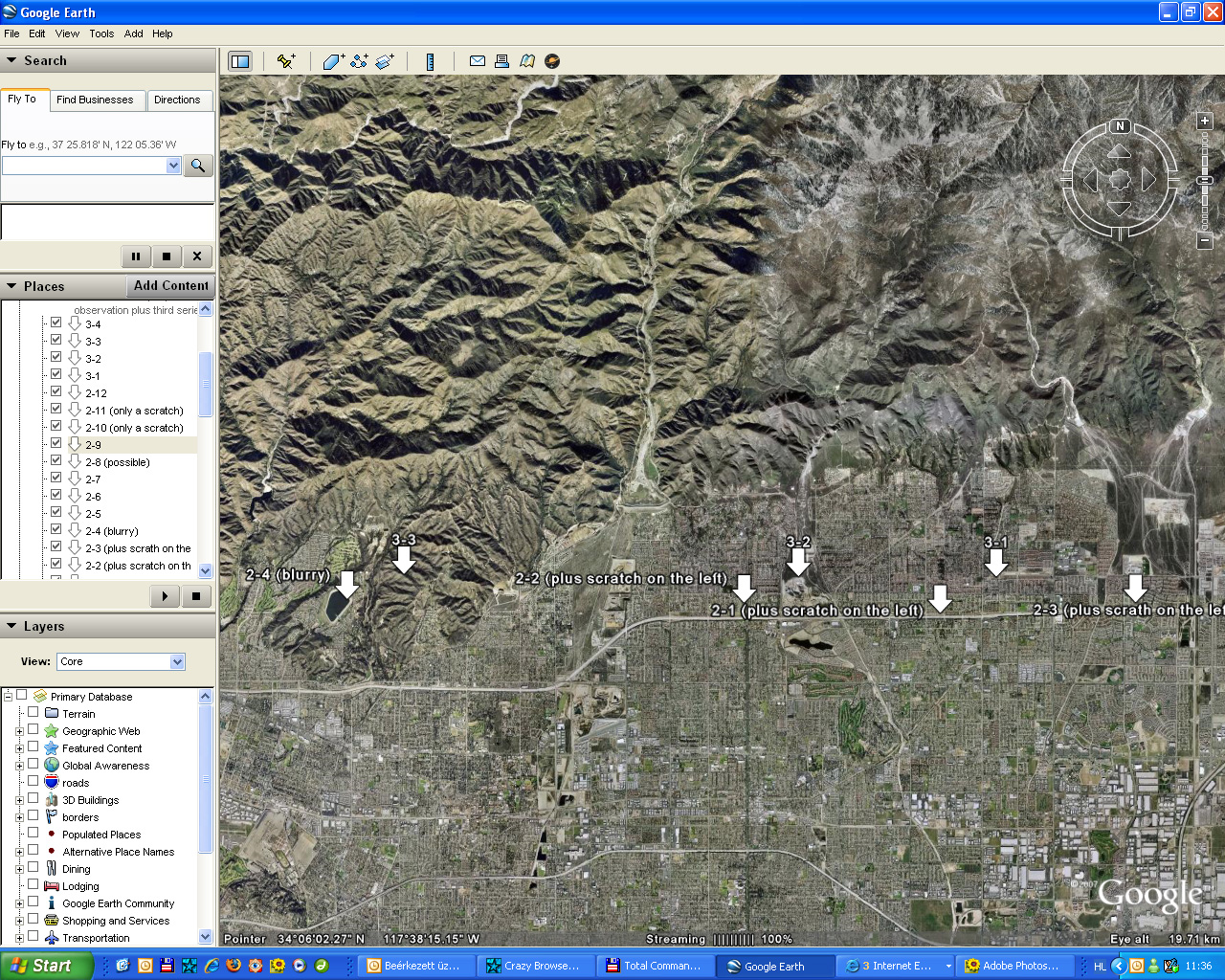The image shows a complex user interface, potentially from a software application or website. At the top, there is a prominent blue rectangle. On the left side of this rectangle, a symbol and some text are visible. On the right side, there is a series of small, outlined squares: a blue square with a white outline, another similar blue square featuring two smaller squares within it, and an orange square with an 'X' in it.

Below this, there is a cream-colored rectangle with some text on the left side. Directly under this, there is a gray rectangle with a downward-pointing arrow and the word "Search." Just below this search bar, several tabs are present but their labels are too small to discern. One of these tabs is attached to a white rectangle containing text. Adjacent to it is a blue-outlined white rectangle with no text, another downward arrow, and a gray square with a magnifying glass icon.

Further down, there is a dark gray horizontal line and another line running vertically. Below these, the section displays a range of colors including cream and greenish hues. On the right side, there is a gray rectangle with two lines inside, a rectangle with a square, and one with an X. Below this setup, another gray rectangle features a downward arrow and the word "Places," with another gray rectangle inside saying "Add Content." Underneath, there is a cluster of folders and downward arrows, but the text is too small to be legible.

Further down the layout, another cream-colored rectangle houses a variety of gray rectangles with different symbols, one pointing right, one with a black square, and another with a downward arrow labeled "Layers," followed by more unreadable text. Alongside this panel, there is a topographical map adorned with arrows pointing towards the center.

Near the bottom left, a green Start button with the Windows symbol and the word "Start" in white is present. Flanking this button are blue rectangles featuring various symbols and text. These are arranged in a pattern that alternates between darker and lighter blue. Additionally, there is a darker blue rectangle marked with an 'H', a blue circle containing a left-pointing arrow, a yellow square, and a green person symbol, among other indistinct symbols and characters.

This detailed, intricate layout suggests a sophisticated interface filled with numerous interactive elements and tools.